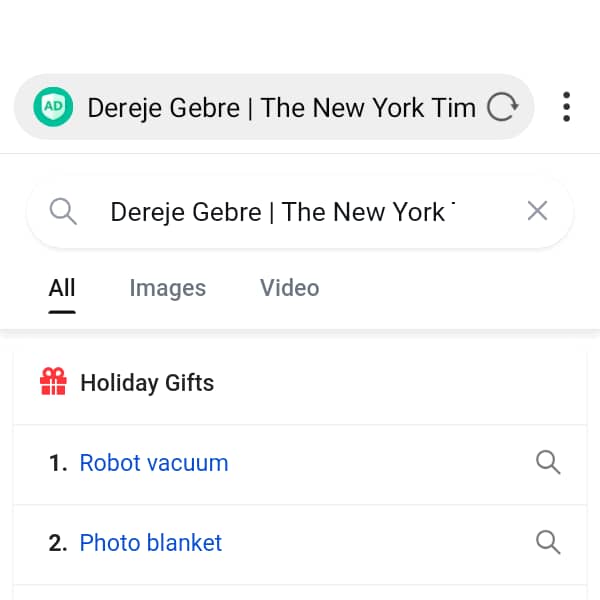The image depicts a webpage on a search engine platform resembling Google, displayed against a white background. At the top, the address bar features a green ad blocker shield icon, indicating an ad blocker is active. Next to the icon, the text "DEREGEBRE" appears in black font, followed by a vertical line and the partially visible text "The New York Tim," suggesting the full text should be "The New York Times." To the right of this, there is a refresh icon and a vertical three-dot menu for additional options.

In the main search bar below, the query "DERGEBRE the new New York" is shown, with a small ‘X’ icon to clear the search. Below the search bar, there are options to filter results by "All," "Images," or "Videos," with "All" currently selected. 

Beneath these options, a promotional section showcases holiday gift ideas. The first item is described as "Number one, robot vacuum," accompanied by a blue clickable button labeled "robot vacuum" for further search results. The second item on the list is "Photo blanket," also featured as a link in blue text, allowing users to search for "photo blanket" with a single click.